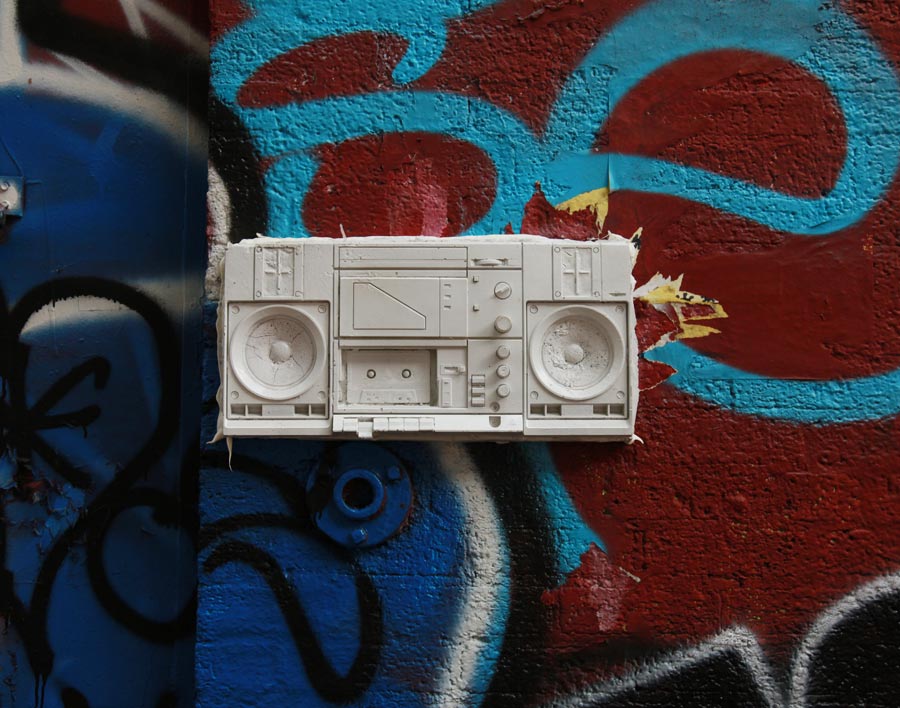The image depicts a dismantled, old-fashioned, plastic boombox, prominently positioned against a graffiti-covered brick wall. The boombox, missing its cover and with the play button engaged, showcases a cassette still inserted in its deck. It features multiple knobs and two large speakers flanking either side of the cassette deck. The surrounding alleyway ambiance includes a wall and a door, both elaborately spray-painted in a palette of powder blue, navy blue, red, wine, white, and black. The intricate graffiti designs and lettering, though unreadable, add a vibrant, chaotic backdrop to the solitary object in the scene. No people or animals are present in the photograph.